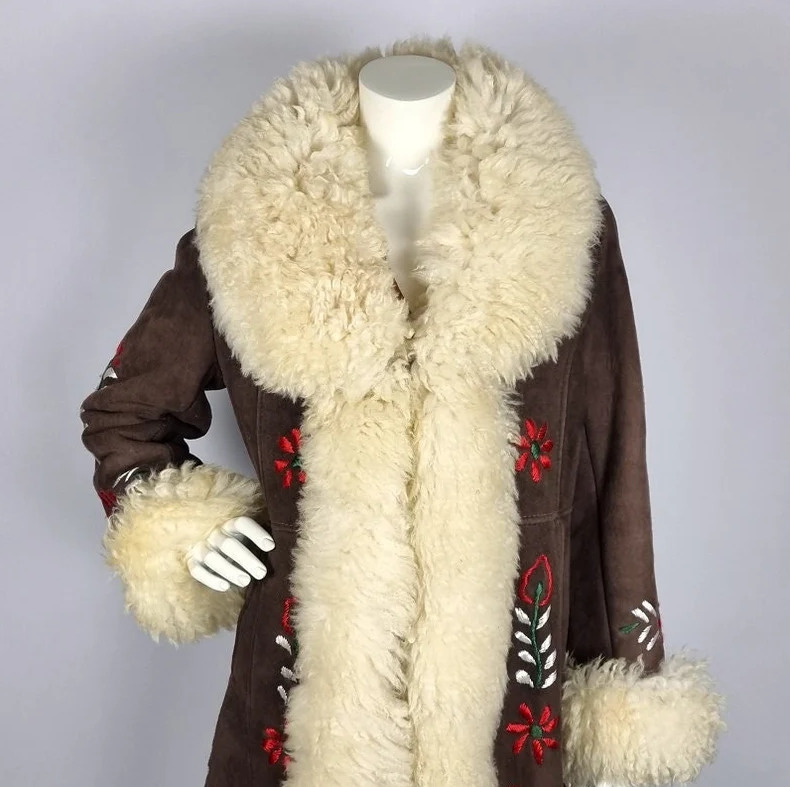This photograph captures a detailed image of a headless white mannequin adorned in a striking long coat. The mannequin stands against a grey wall, with its right arm casually placed on its hip and the left arm hanging down. The dark brown coat, reminiscent of the stylish Penny Lane coat from "Almost Famous," is crafted from a leathery or possibly suede material. It is richly decorated with intricate white and red floral embroidery along the bottom and sleeves. The coat's most prominent features are its luxurious beige fur linings, which envelop the thick collar and appear at the cuffs, adding a touch of opulence to the overall design.